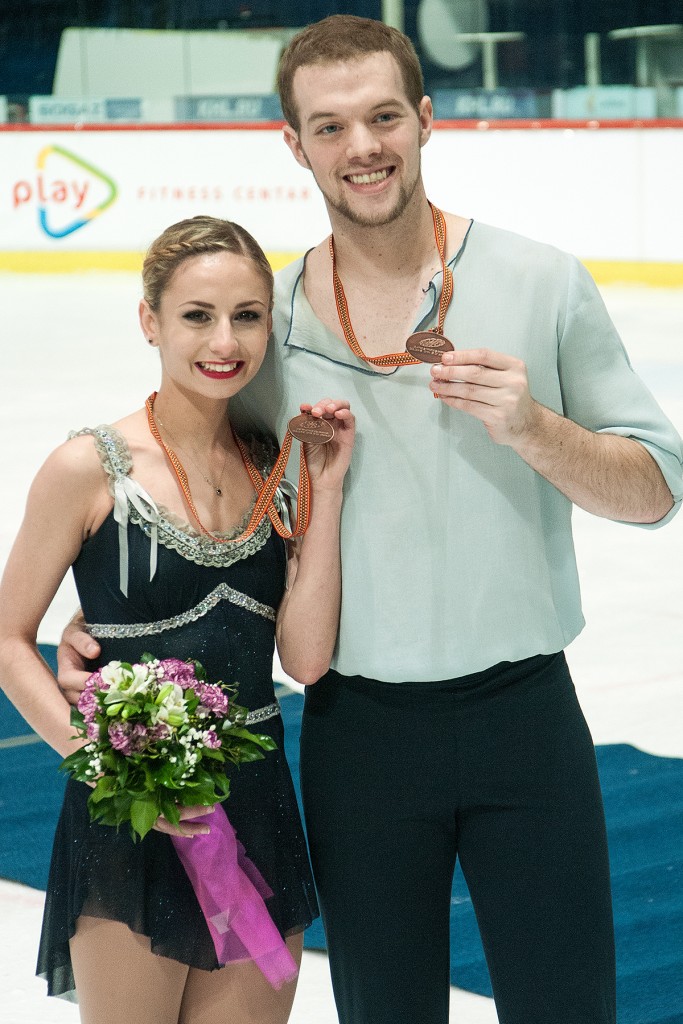The photograph captures a vertically-aligned, celebratory moment featuring a young ice-skating duo at an indoor ice rink. The woman on the left is a short, young skater with light blonde hair braided to the side, cascading over her shoulder in a ponytail. She dons a sparkly, black and silver, short dress and smiles brightly with red lipstick on. In her left hand, she proudly holds up a gold or bronze medal, while in her right hand, she cradles a bouquet of flowers adorned with purple petals, green leaves, and a purple ribbon. 

Beside her stands a man, his arm affectionately wrapped around her waist. He sports short brown hair and thin facial hair, beaming with joy. He wears black pants and a light green shirt with sleeves cut off at the elbows, giving it a minty freshness. He, too, holds up a matching medal. 

The setting is unmistakably an ice rink, with the ice visible beneath them and a distinct background featuring glass panels above bordered partitions in red and yellow. Though partially obscured, the signage reads “fitness center,” marking the location of their triumphant performance.